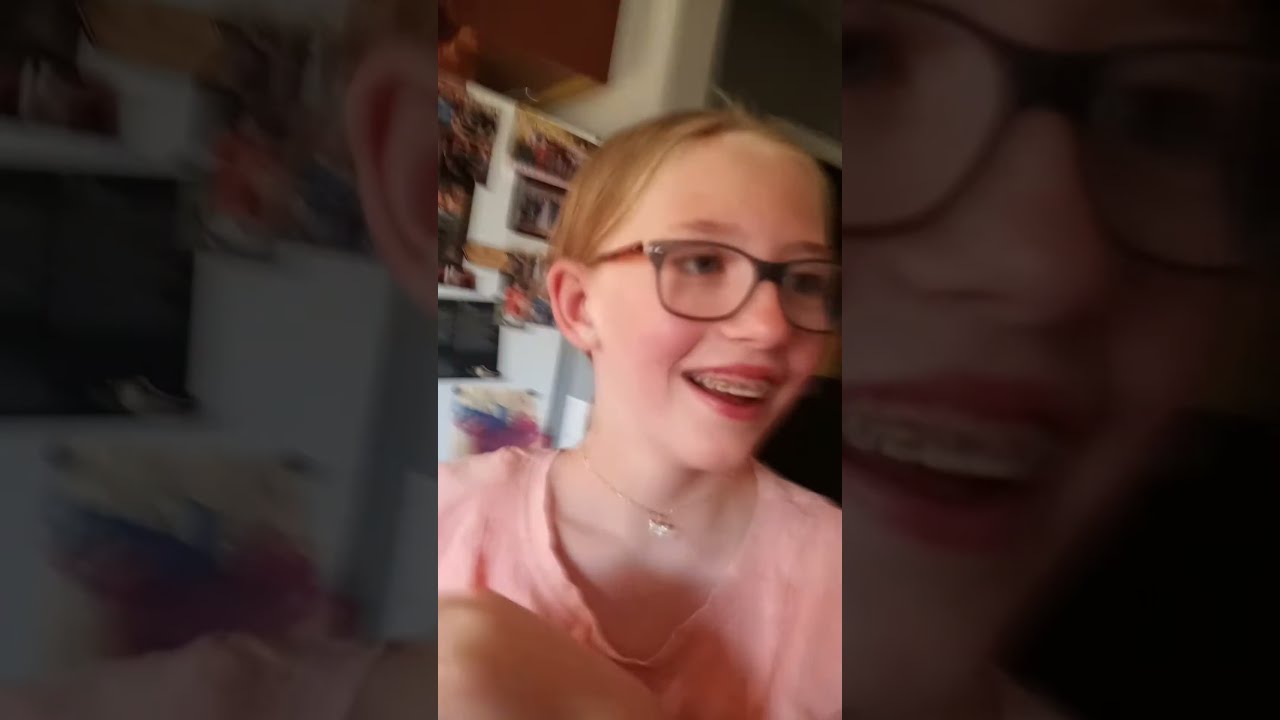The photograph features a young girl, approximately seven to ten years old, with short, strawberry blonde hair. She is smiling, revealing her braces, and is wearing large, dark brown Wayfarer-style glasses. Her attire includes a faded pink shirt with a loose, stretched-out neck and a delicate gold necklace adorned with a shiny butterfly pendant. The image is slightly tilted clockwise and predominantly focuses on her, placing her near the center. In the background, there is a collection of family photos, including a wedding photo and group portraits, along with various artworks pinned to the wall. The setting appears to be indoors, likely in her home, with blurred areas on the sides forming a semi-transparent border. The colors in the image range from pink, tan, and silver to red, brown, purple, blue, white, black, and orange. Additionally, a refrigerator with several pictures on it and a vertical beam are discernible behind her. The photo seems to be a screenshot taken from a mobile device.